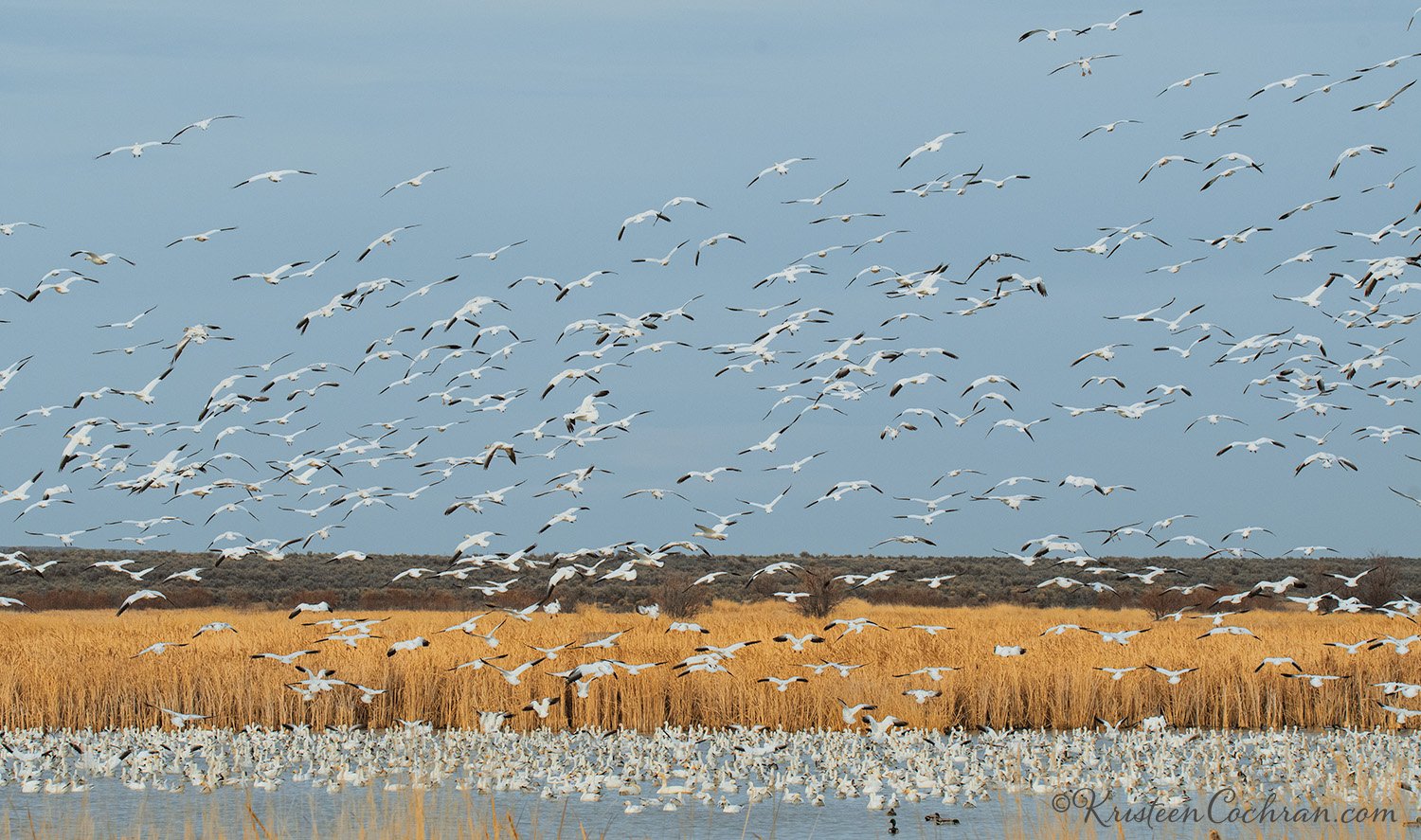This outdoor daytime photograph captures a bustling scene in what appears to be a semi-watery, farm-like field filled with dense, yellowish-brown vegetation. The field, possibly a cornfield, is teeming with hundreds, if not thousands, of birds. These birds, mostly white with black wingtips, are both in flight and standing around, with many floating on the water’s surface in the foreground. The sky above is a clear blue, slightly hazy with some clouds. In the distance, short trees can be seen, adding depth to the landscape. A small pond surrounded by tall, muted green, and bright brown grass can also be seen, indicating the semi-watery nature of the area. In the bottom right corner of the image, there is an unclear watermark from a website, possibly reading “Kitch.” The birds dominate nearly the entire picture, except for a small area in the upper middle part of the image.